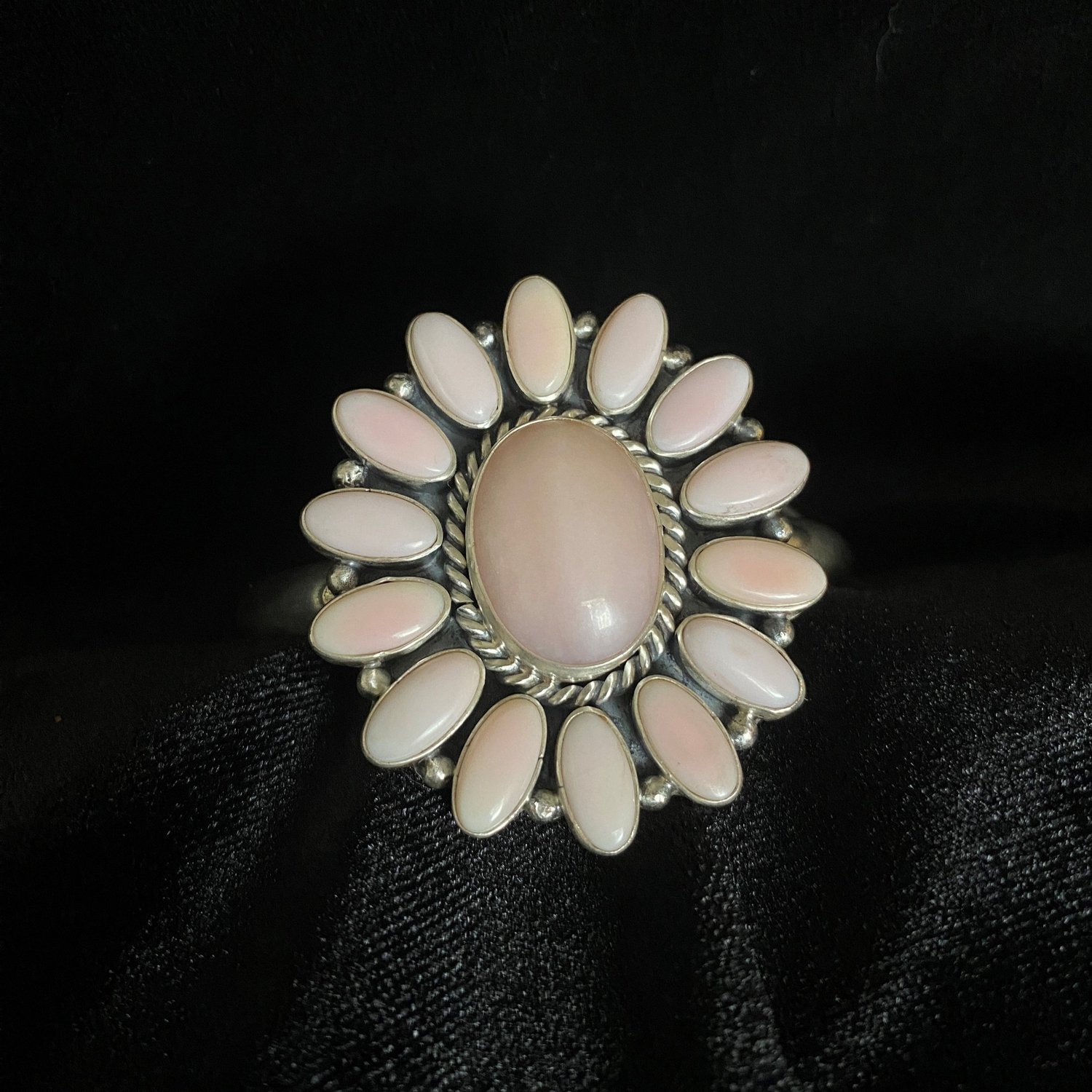The image presents a close-up view of an intricately designed brooch, set against a black fabric background. The focal point of the jewelry is a large, elliptical pearl-like gem that exhibits a polished, white sheen with subtle hints of pink and green reflections. This central gem is encircled by a metallic decoration, possibly made of pewter or silver, featuring a rope-like design. Radiating outward in a circular pattern are approximately 15 to 20 smaller, elliptical stones of a similar pearl or ivory material, arranged to resemble the petals of a flower. Each of these petal-like gems is accentuated with a small metallic ball placed between them, creating a harmonious and detailed floral motif. The brooch is meticulously crafted to highlight the contrast between the lustrous gems and the intricate metallic elements, all beautifully showcased on the black cloth background.